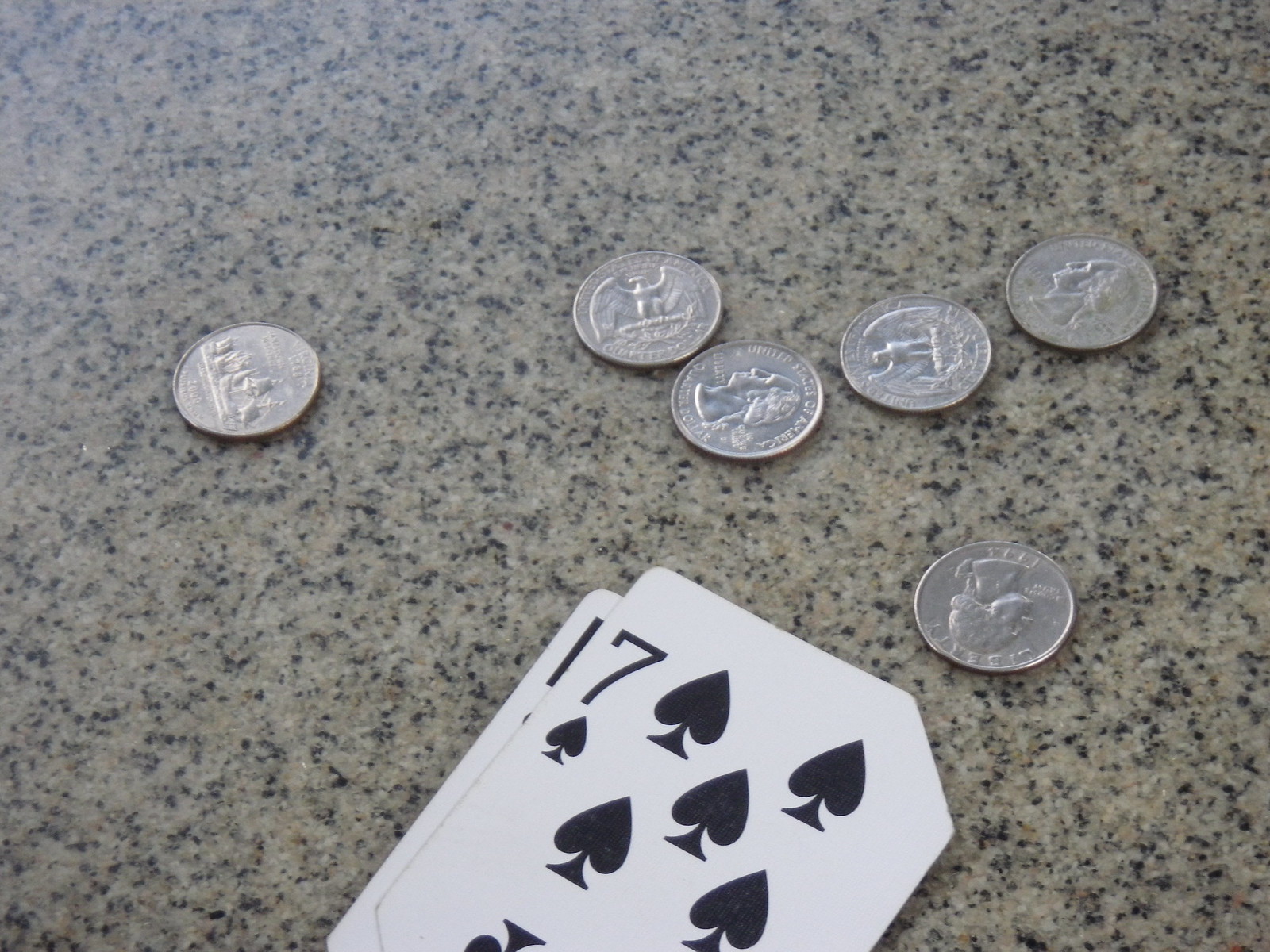The image captures a detailed scene of a granite-like countertop with a speckled tan, black, and brown pattern. At the bottom center of the frame, partially cut off, is a deck of white playing cards, with the top card being the Seven of Spades. This card features a black number '7' and black spade symbols; notably, five spades and part of a sixth are visible.

Scattered across the countertop are six quarters. Three of these quarters display the tails side with two featuring the traditional eagle design, while the third quarter's tails side showcases a unique design with a ship and the text "Virginia," dated 1788-2000. The other three quarters display their heads side. Most of these coins, five to be precise, are clustered together on the right-hand side of the countertop. Notably, the quarter with the ship design is positioned separately on the left side of the image.